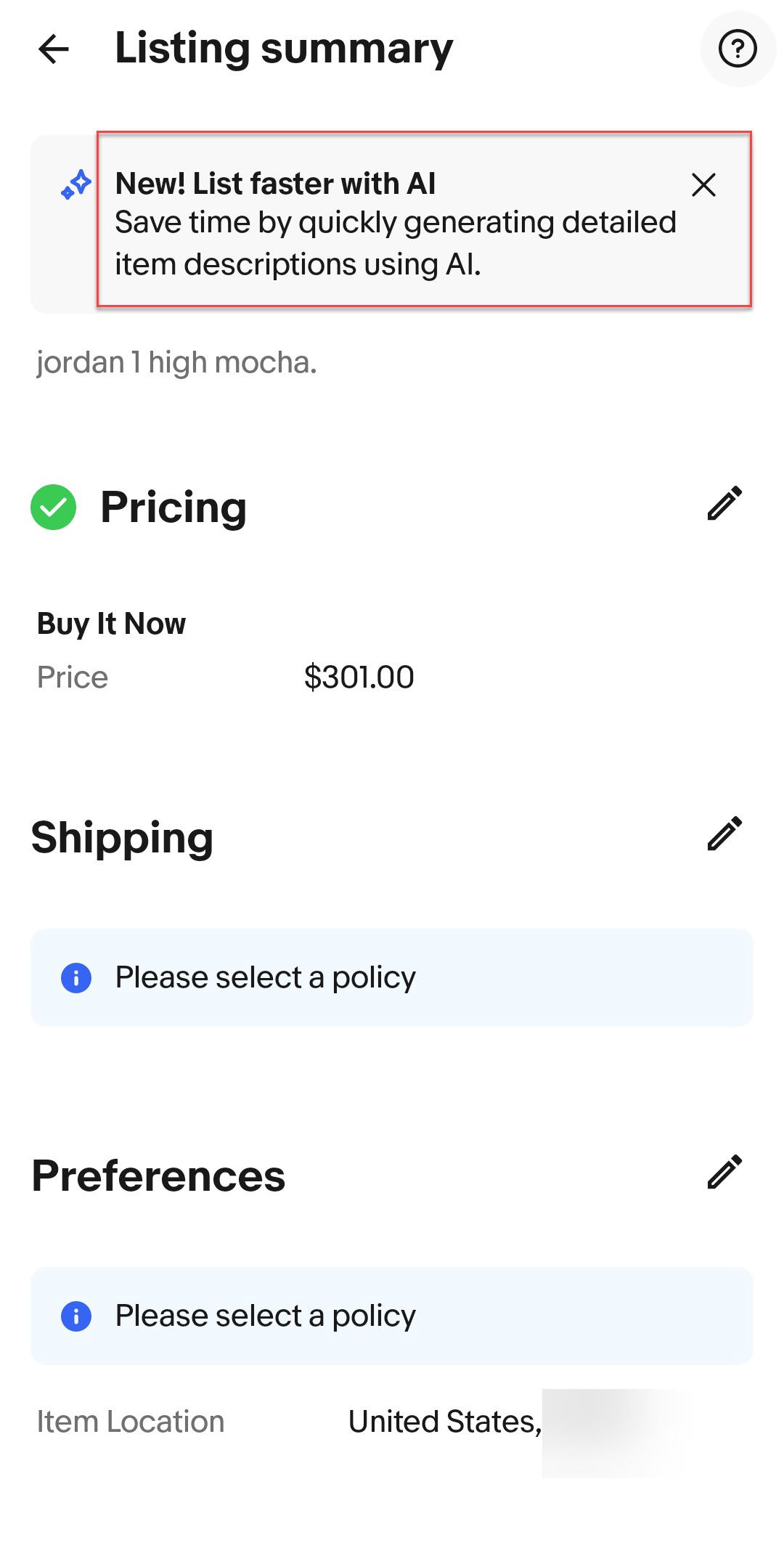The image depicts a website interface where a person is in the process of purchasing an item priced at $301. At the top of the interface, there is a listing summary and a back arrow located in the top left corner. In the top right, a question mark inside a circle is present for additional help. Below this, a tab reads, "New: Listen faster with AI. Save time by quickly generating detailed item descriptions using AI."

Underneath this tab, a green circle with a check mark symbol indicates the pricing section, accompanied by a pencil icon for editing. The buy now price is clearly stated as $301. Following this, there is a section for shipping details, with another pencil edit icon situated on the right side. Beneath the shipping section, a blue tab is labeled "Select a Policy," and next to it is a blue circle containing an "i" for information.

Further down, another section titled "Preferences" also features a blue tab with an "i" symbol, indicating the option to select a policy for preferences. To the right of this, an identical pencil edit symbol is present. The item location is specified as the United States, with an additional location that is blurred out. The website has a predominantly white background with black text for most of the descriptive details.